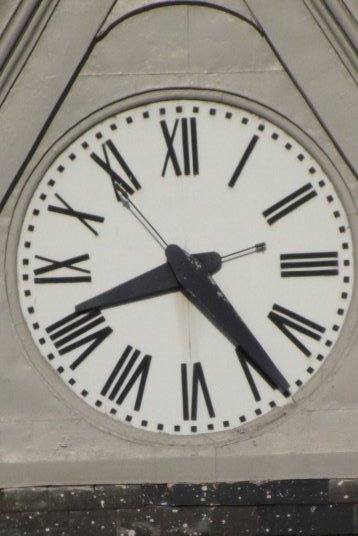A striking black and white close-up of a majestic clock mounted on a historic building. The clock's large, round face, adorned with Roman numerals, stands out prominently. The thick black hour and minute hands point to approximately 8:24, while a thin second hand ticks away. The upward angle of the shot provides a compelling perspective, highlighting the clock's elevated position on the textured façade. Surrounding the clock is a rounded, cylindrical design suggesting an architectural element, possibly concrete, adding to the clock's grandeur. Below, a darker brick ledge—speckled with white spotting—contrasts sharply with the clock face. Minute markers, denoted by small black rectangles, encircle the numerals, adding to the detailed craftsmanship of this timeless piece.